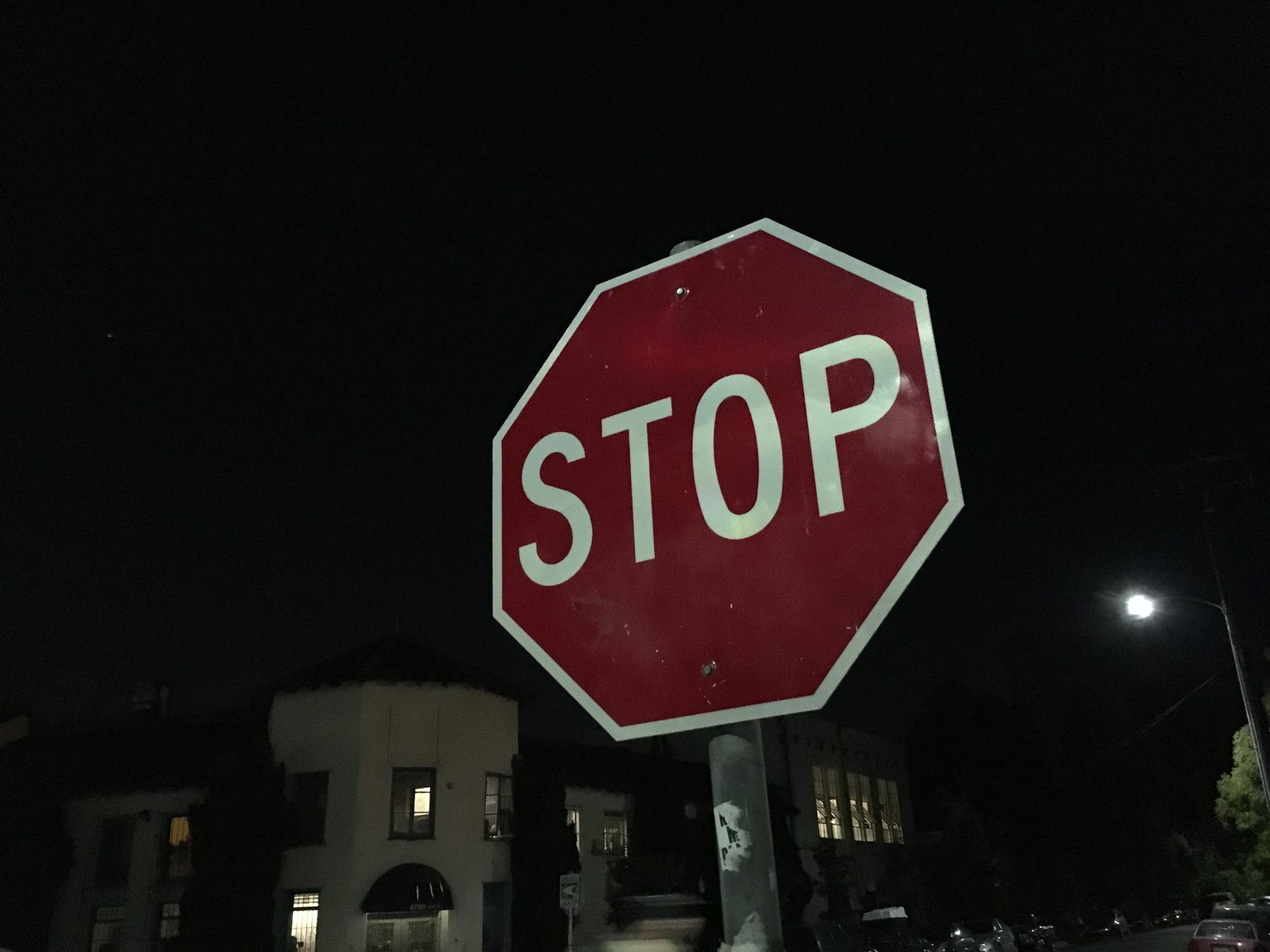The digital photograph captures a night scene dominated by an inky black sky, suggesting it was taken long past sunset. At the center, an octagonal red stop sign with a distinct white border stands prominently, bearing the word "STOP" in bold white capital letters. The sign is securely attached to a silver metal pole with rivets and shows remnants of peeled stickers on its surface.

On the right side, a lit lamppost casts a soft white glow, partly illuminating the scene. Nearby, green leaves of a tree poke out from the darkness. On the left and right sides of the image, cars are densely parked along the street, lined with a mix of residential buildings.

The most notable building, situated on the bottom left, is primarily white with a contrasting dark roof. It features large windows allowing some indoor light to spill outside. The building's frontage includes a three-sided corner, a window on the bottom left that's brightly lit, and a small canopy over the front door. Additionally, a sign is affixed to the steps leading to the entrance.

In summary, the photograph captures a tranquil nighttime street scene with a prominent stop sign, softly illuminated surroundings, and detailed elements of an urban residential setting.